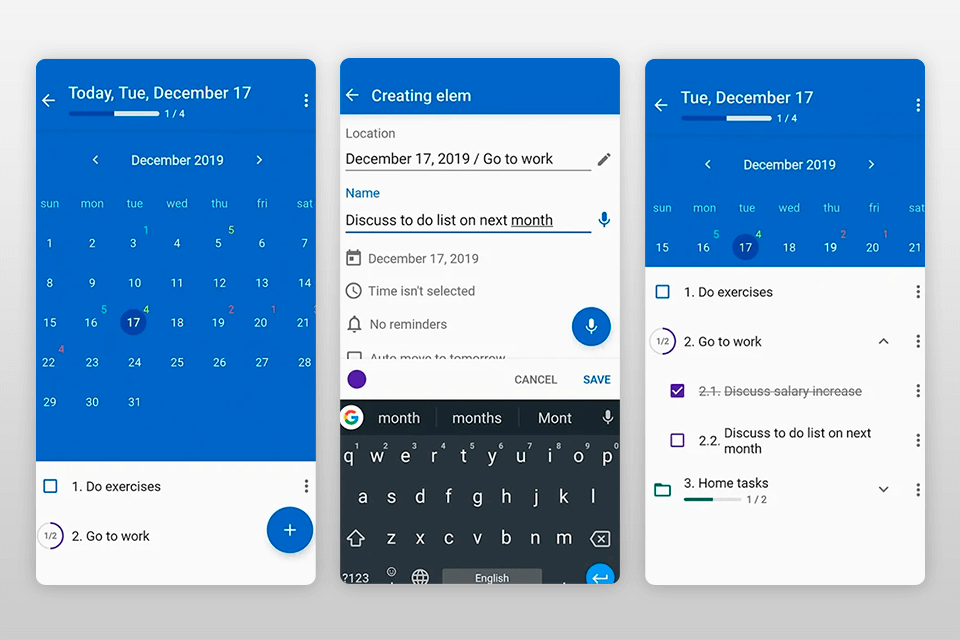This image is a composite of three smaller images displayed within a rectangular frame. 

1. **Top Section**: This part shows a digital calendar set to Tuesday, December 17th, 2019. The date is clearly marked, and the day's agenda includes tasks such as "do exercises" and "go to work."

2. **Middle Section**: The second picture appears to be a task creation interface screen. It shows the task "Creating LM" scheduled for December 17th, 2019, with a note to "discuss to-do list for next month." The time for this task is not specified, no reminders are set, and a keypad is visible on the screen, indicating that this is a currently active input form.

3. **Bottom Section**: The final image once again highlights the date, Tuesday, December 17th, 2019, along with a to-do list for the day. The options include "do exercises," "go to work," "discuss to-do list on next month," and "look at home tasks."

Each of these images contributes to a comprehensive overview of the day's schedule, detailing the tasks, their context, and the tools being used to manage them.